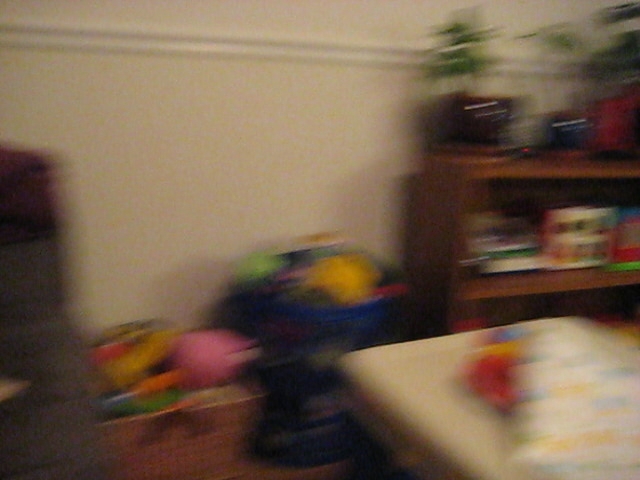This is a very blurred photograph depicting what appears to be a children's bedroom or playroom. The image shows various items lined up against a white wall with white molding about six feet high. Central to the scene is a blue cylindrical container brimming with brightly colored toys, including notable yellow and green items. Adjacent to it is a whisker basket filled with more toys, and a wooden toy chest that also contains assorted toys, with prominent colors like pink, orange, blue, and yellow.

On the right side, there is a beige plastic table scattered with red, yellow, and blue toys, and nearby are two tubs full of colorful playthings in pink, yellow, green, and blue hues. A lone figure wearing gray is vaguely outlined towards the left of the image. In the center-right of the photograph, there is a low, light brown bookshelf or entertainment stand. This piece of furniture holds toys resembling buildings, colored white and red, and is topped with dark blue vases accented with brown, containing dark green leafy plants. Additionally, there are shelves with potted plants and an assortment of books. There’s also a small bed or something similar visible towards the right-hand corner, adding to the impression of a child's room. Despite the overall blur and indistinctness of the photograph, the playful and colorful elements suggest a lively and engaging space for a child.